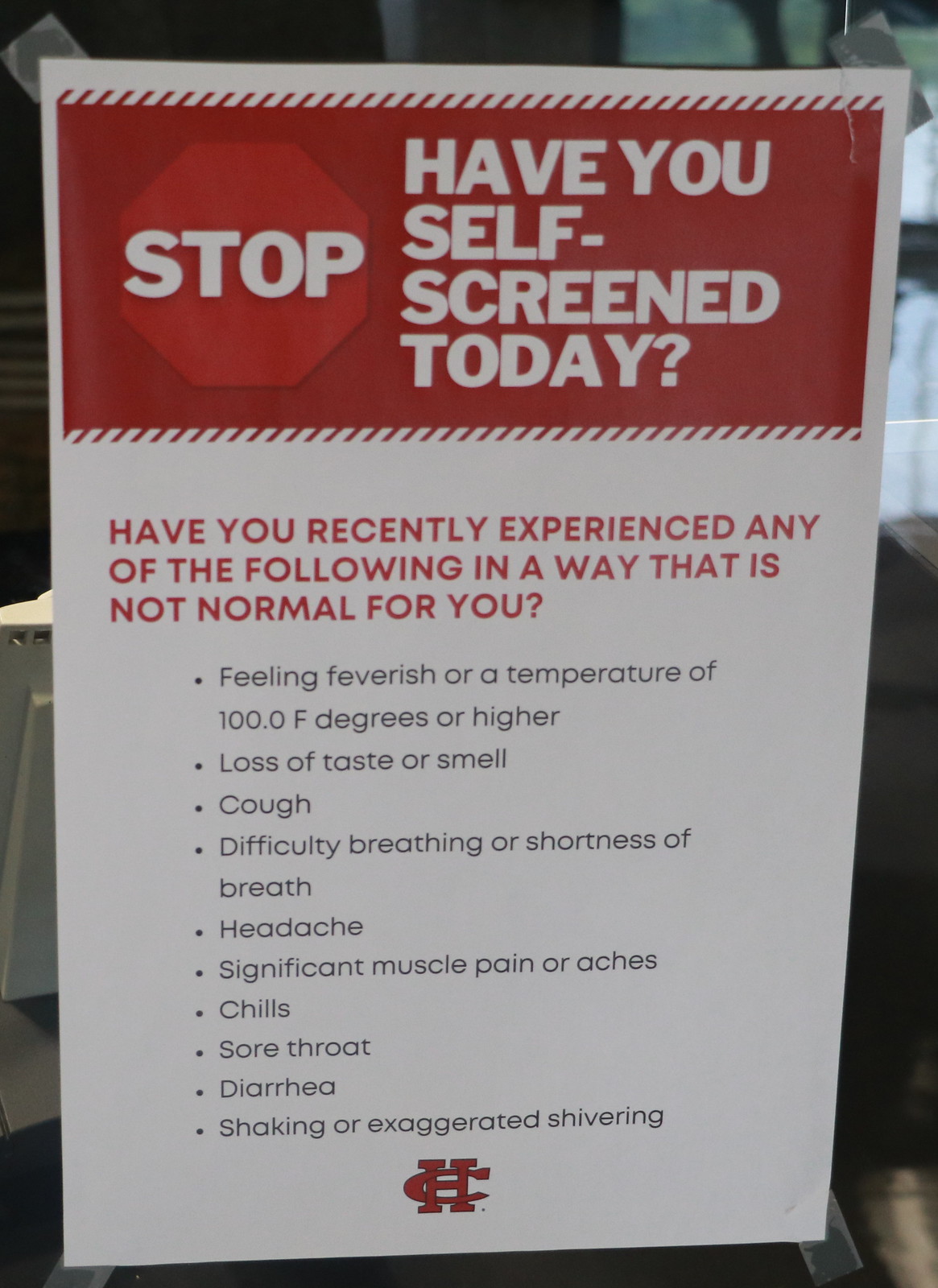This is a vertical rectangular poster taped to a glass window, possibly in an office setting, as evidenced by the visible desks, chairs, and computer equipment in the background. The poster is affixed with cello tape at all four corners. It features a prominent red rectangle at the top, with a stop sign on the left side displaying the word "STOP" in big white letters. To the right, also in big white letters, is the question "Have you self-screened today?" 

Below this red rectangle, the rest of the poster has a white background with a subheading in red, capitalized letters that reads: "Have you recently experienced any of the following in a way that is not normal for you?" Underneath this, in black letters and organized into bullet points, are symptoms including:

- Feeling feverish or a temperature of 100.0°F or higher
- Loss of taste or smell
- Cough
- Difficulty breathing or shortness of breath
- Headache
- Significant muscle pain or aches
- Chills
- Sore throat
- Diarrhea
- Shaking or exaggerated shivering

At the bottom center of the poster, there is a logo composed of a red combination of the letters "C" and "H".